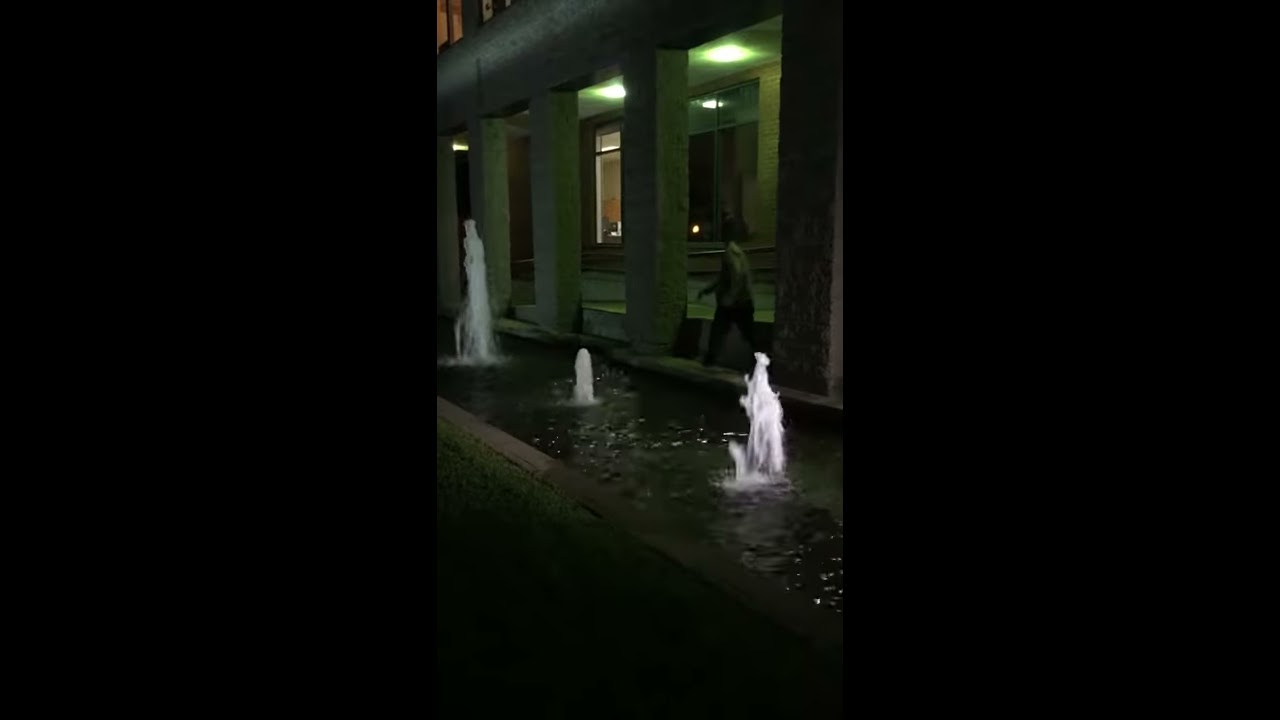The photo captures a nighttime scene outside a large stone building, characterized by its geometric architecture and subtle lighting. Dominating the scene are five rectangular gray columns, which extend vertically from a concrete floor and are topped by another concrete slab, angled slightly. The atmosphere has a somber, dark quality, accentuated by hues of green reflecting off the lower portion of the scene. Nestled between these columns and a green lawn area is a rectangular water fountain, where three small jets of water burst upward, creating delicate arcs of white spray. Behind the columns, windows are visible, softly illuminated, suggesting an active nocturnal ambiance inside. A lone figure, discernable by a white shirt and possibly black pants, walks between the columns, adding a touch of human presence to the otherwise still and structured landscape.